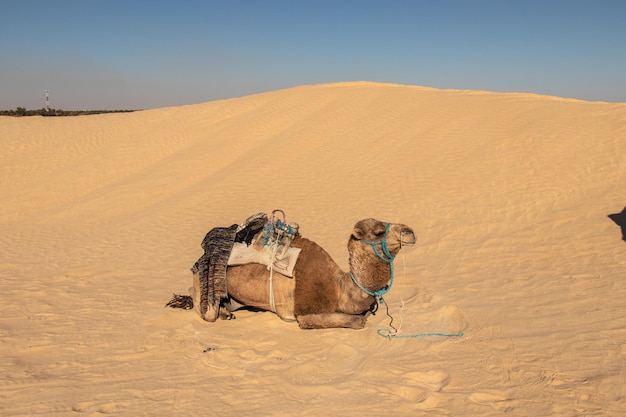The photograph depicts a camel lying down in the desert, specifically on a yellow sand dune, with its legs tucked underneath it. The side profile shows the camel facing to the right with its tail end to the left. The camel is equipped with an aqua green collar around its face and neck, and carries a distinctive harness that appears to contain medical equipment or a unique saddle featuring a bar on top for gripping. A woven blanket in shades of brown and a tan quilted blanket are draped over and under this contraption. The forepart of the image shows disturbed sand around the resting camel, suggesting movement or wind. In the background, the top quarter of the image is dominated by a clear blue sky, with a faint presence of greenery, possibly sagebrush, on the distant left side creating a subtle brown tint due to wind-blown sand. Additionally, there is a shadow of an unidentified object in the right part of the image, adding a mysterious element to the scene.